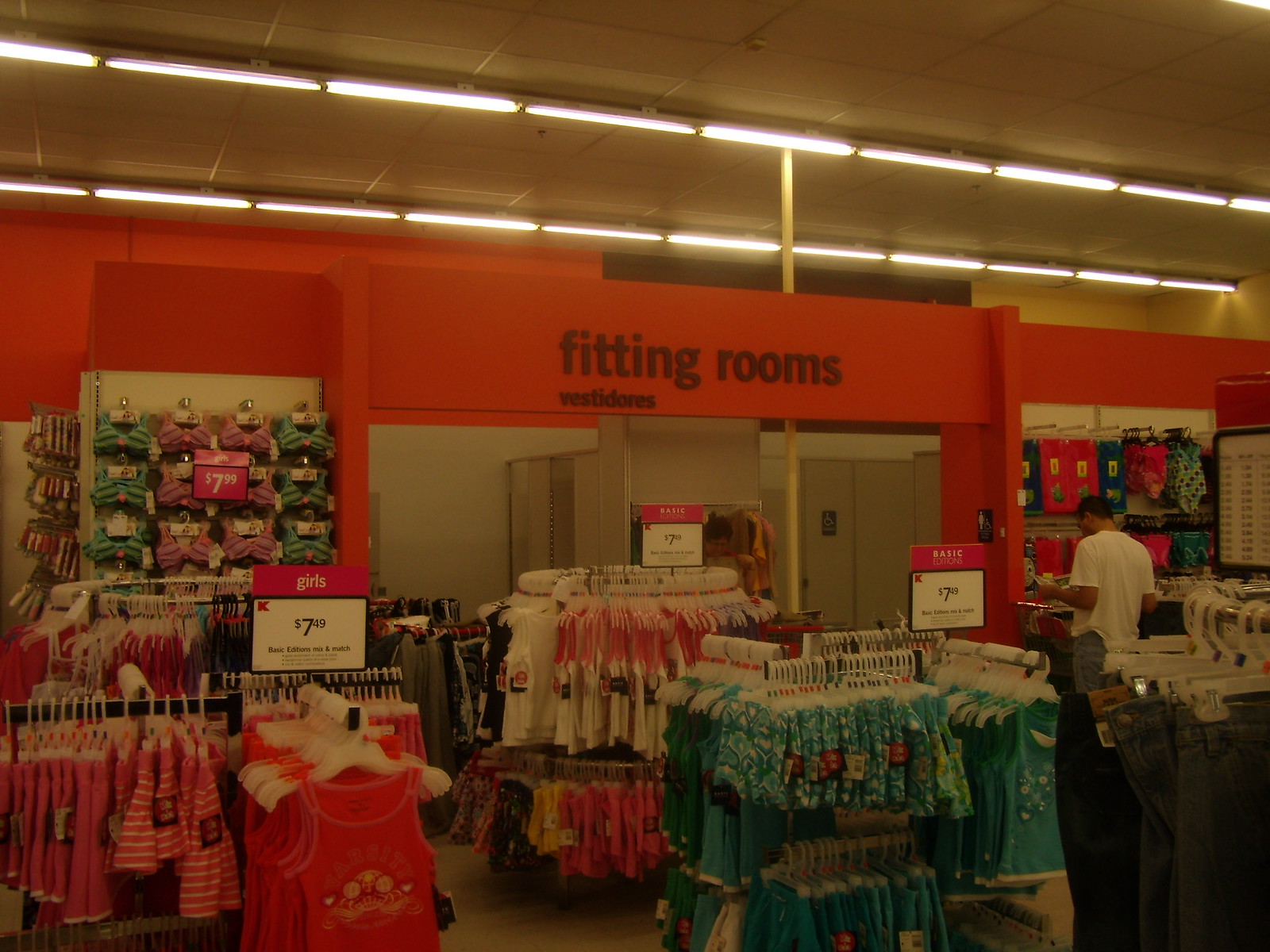The photo depicts an indoor store setting with a prominent wall in the background painted a light red color, labeled "Fitting Rooms" in black text, with a Spanish translation below it. The ceiling features two rows of fluorescent lights. Beneath and around the "Fitting Rooms" sign, shelves display assorted clothing, including colorful bathing suits and children's clothes, with signs indicating categories such as "girls" and "basic edition" alongside price tags. The fitting rooms themselves are visible behind the shelves, some equipped with handicap signs suggesting larger spaces. In the foreground, there are several racks of clothes organized by color schemes, including stacks of green clothing, white shirts with red accents, and red items on the far left. On the right side of the image, a man in a white T-shirt and blue jean shorts is browsing products on a shelf, while a woman is seen holding something up to a mirror. Additionally, a yellow pole is noted in the background of the fitting room area, adding to the structural details of the scene.